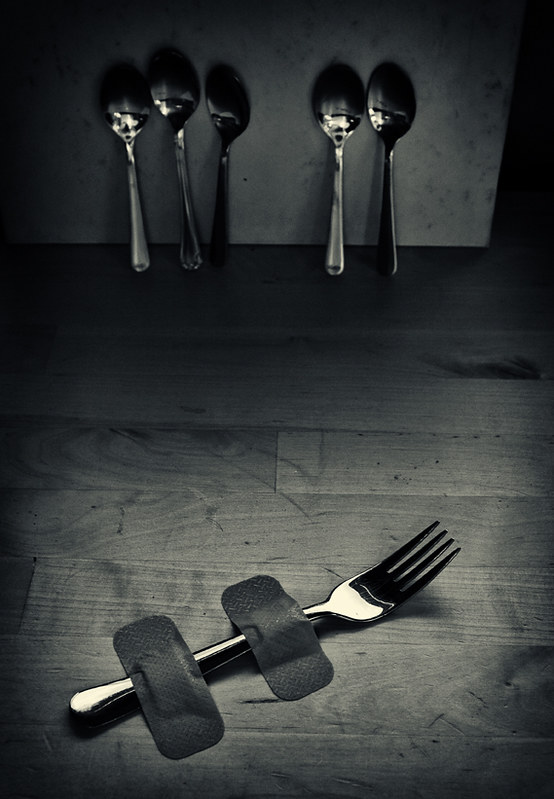This monochrome photograph, possibly with a slight sepia tint, captures a dark and gritty scene featuring silver-toned cutlery arranged on a rustic, distressed wooden floor. The photograph is vertically oriented, and the edges are shrouded in deep black shadows, enhancing the spotlight effect on the central subjects. At the top of the frame, leaning against a textured ivory or white wall, are five reflective spoons arranged into two groups—three on the left and two on the right, with a small gap between them. The concave surfaces of the spoons face the viewer, reflecting light in the otherwise low-lit image. In the foreground, a silver fork lies diagonally, its prongs pointing upward towards the right-hand corner. The fork is restrained by two dark band-aids affixed across its handle, evoking the imagery of a hostage scene. This arrangement, with the attentive spoons and the pinned fork, creates an almost theatrical tableau, rich with implied narrative and dark humor.